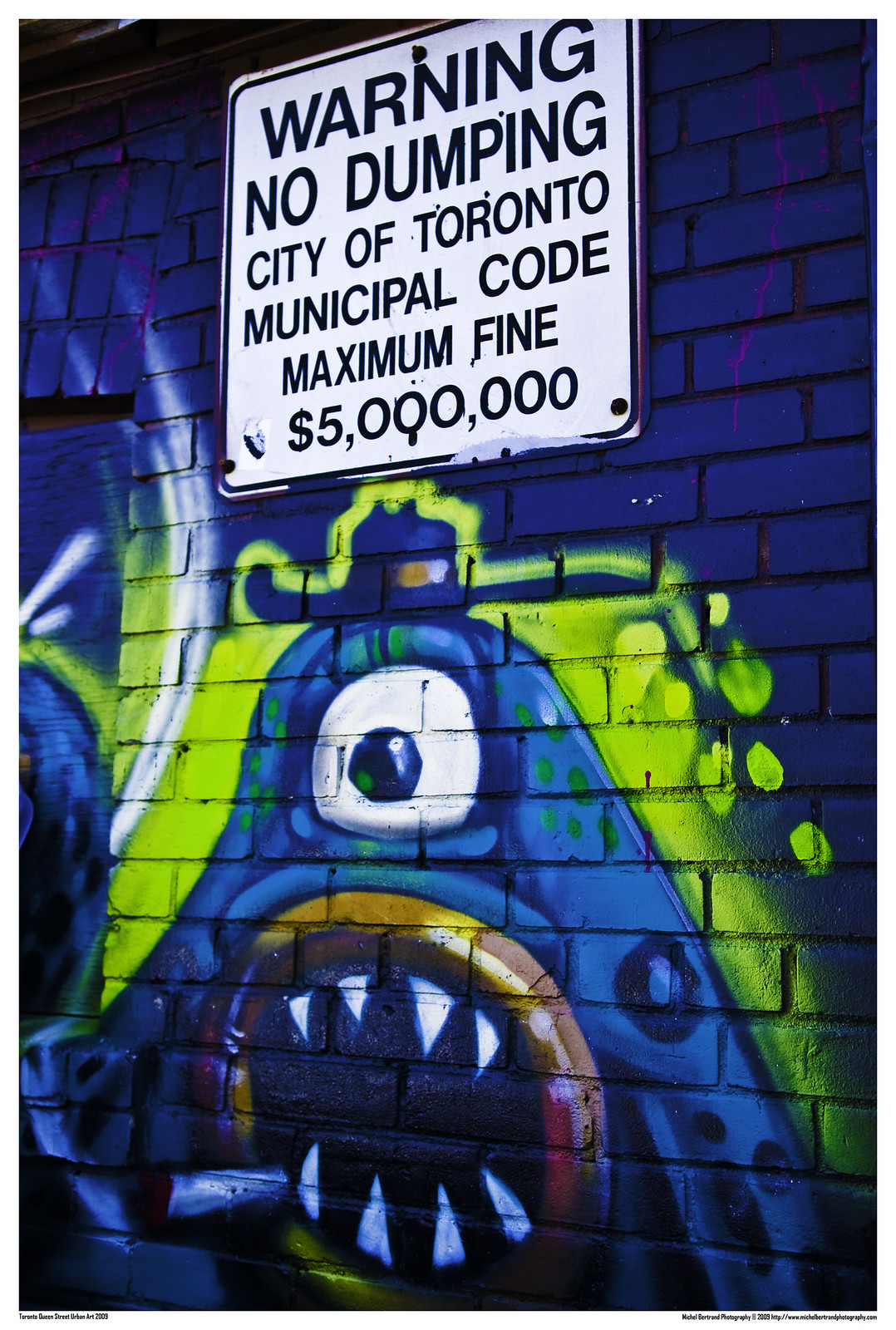The photograph depicts a brick wall painted blue, adorned with vibrant graffiti of a one-eyed monster. The monster, which has green spots and is surrounded by a green background, is characterized by its single large eye and a mouth that is a perfect circle outlined in red, featuring two rows of four sharp, spiky white teeth each. The monster is also wearing a large-brimmed blue cap. Above this detailed graffiti is a slightly slanted metal sign with a white background and black lettering. The sign reads, "Warning. No dumping. City of Toronto. Municipal Code. Maximum fine $5,000." This detailed and colorful artwork contrasts sharply with the official tone of the warning sign, creating a unique visual.